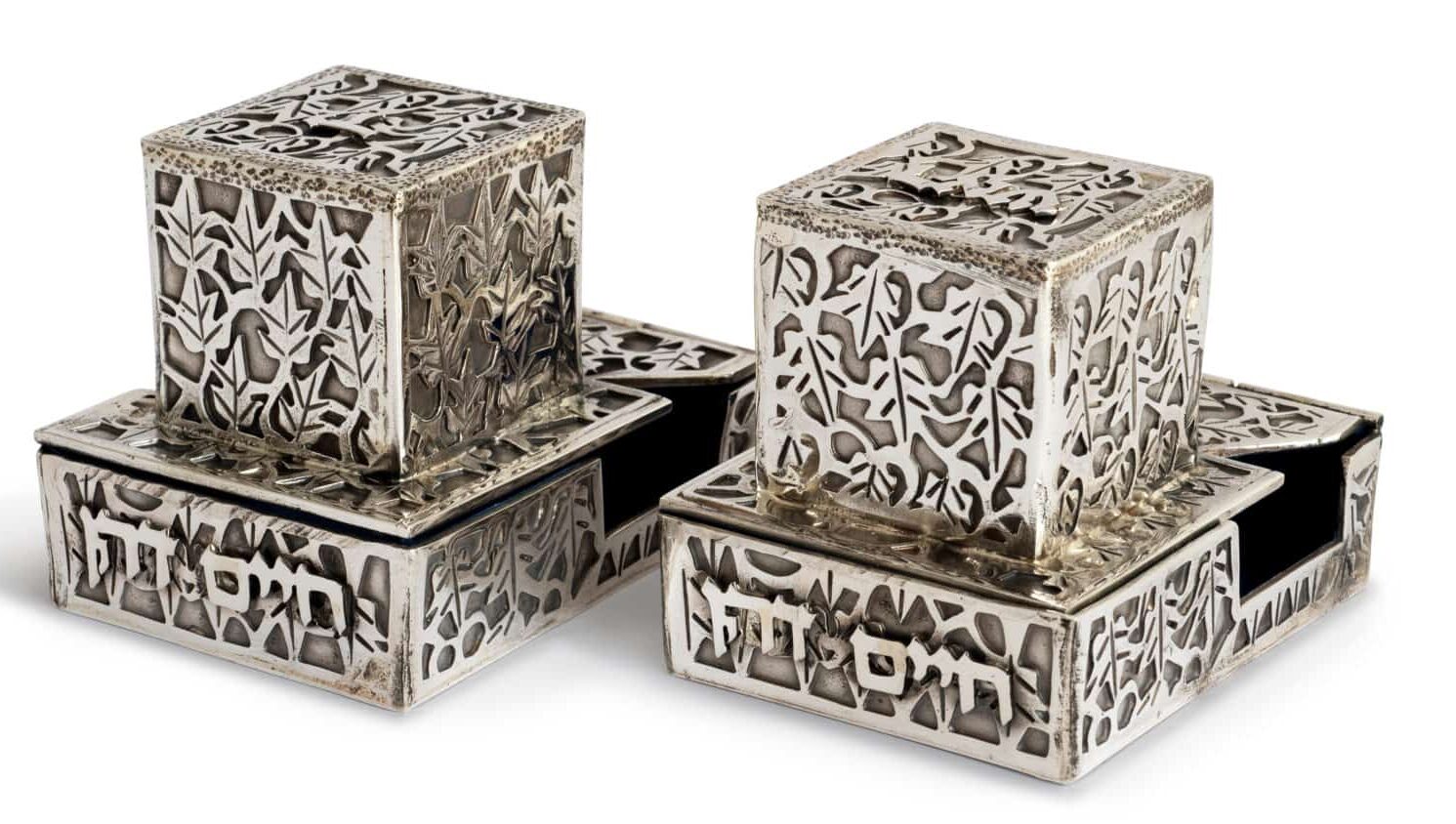In this picture, set against a white background, there are four intricately designed metal boxes. At the bottom, two rectangular, cigar-box-shaped containers sit side-by-side, each with a small squared cutout along their sides where the lids meet. Positioned on top of these rectangular boxes are two smaller square boxes, each meticulously placed towards the foreground of the image and made in the same ornate style. 

All four boxes feature a rich tapestry of carvings and patterns, blending floral motifs, leaf designs, simple geometric shapes, and symbols that resemble a foreign script, potentially Arabic. The detailed craftsmanship suggests they could be used for storing jewelry, Dungeons & Dragons dice, herbs, or other small treasures. The overall silver color of the boxes is punctuated with darker insets, enhancing the elaborate carvings and giving them a luxurious and sophisticated appearance.